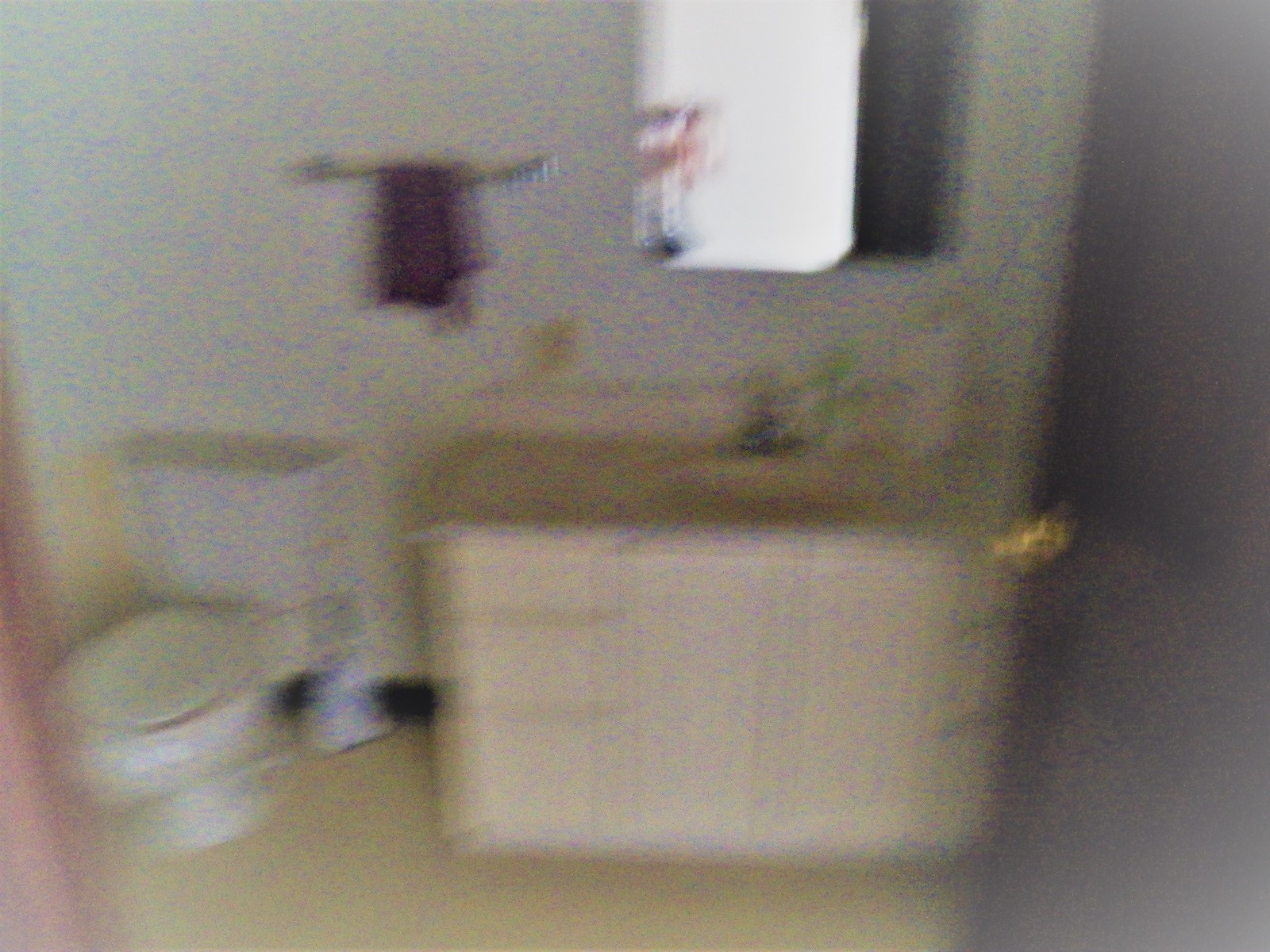A blurry photograph of a bathroom reveals various fixtures and details, albeit with some color and focus inconsistencies. On the left side of the image, there is a white toilet positioned diagonally, facing the lower-left corner. The toilet seat and bowl appear to be a slightly tan hue. Adjacent to the toilet on the right, there is a tan-colored sink with a base composed of both cabinets and drawers. The sink is equipped with three drawers on its left-hand side while the cabinets open below, providing storage. Above the sink, there is a silver faucet and a sizable mirror that captures a partial reflection in its lower-left corner. On the back wall between the toilet and the sink, a towel rack holds a dark-colored, possibly black, hand towel. The overall bathroom setup, though blurry, offers a glimpse into its layout and functional elements.